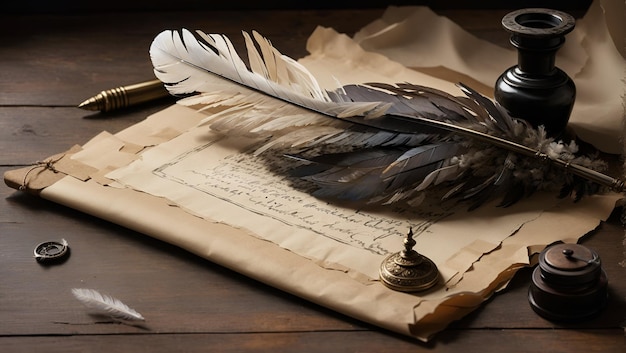A dimly lit photograph depicts an antique scene atop a wooden tabletop. At the center lies a weathered, reddish piece of parchment, ragged at the edges with faint, unreadable script visible at the bottom. Resting on the parchment are two quill pens, one black and one brown, and a small, brass inkwell beside them. To the left of the parchment, there is a small ring glinting subtly in the low light. A bronze ink jar is positioned near the lower edge of the parchment, and a diminutive bell sits quietly in the lower-right corner. A button lies loosely on the table near the parchment's edge. The overall ambiance is steeped in old-timey charm, with a background composed of rich, brown wood, adding warmth and depth to the scene.